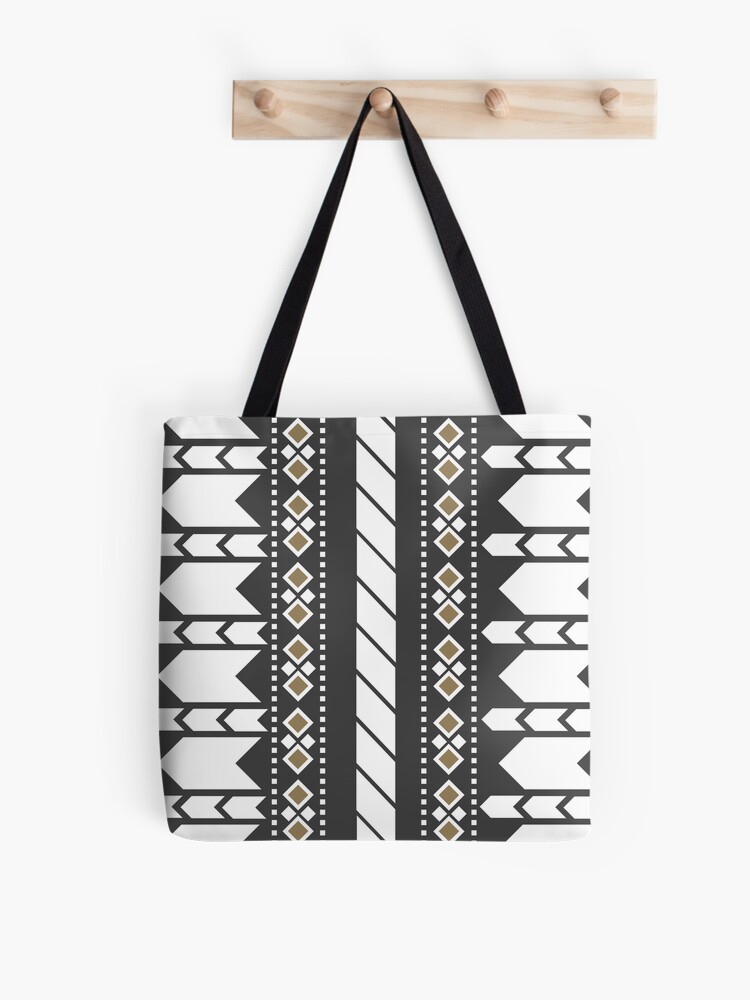The image captures a tote bag with a black strap hanging from the second peg of a wooden peg rack with four pegs, against a white background. The peg rack is crafted from light brown wood. The tote bag features a complex pattern, primarily set against a dark gray to black background. The design includes white and yellow-beige geometrical elements, such as diamonds, parallelograms, and trapezoidal shapes. The central vertical stripe of the tote has thin black lines dividing it into segments with around ten visible lines. Adjacent to this stripe are white diamonds with light red centers, flanked by additional white dots. On the left and right sides of the bag, the pattern forms shapes reminiscent of arrows pointing left, formed by sandwiched parallelograms creating black triangles at their bases. The intricate design is reminiscent of Native American art.